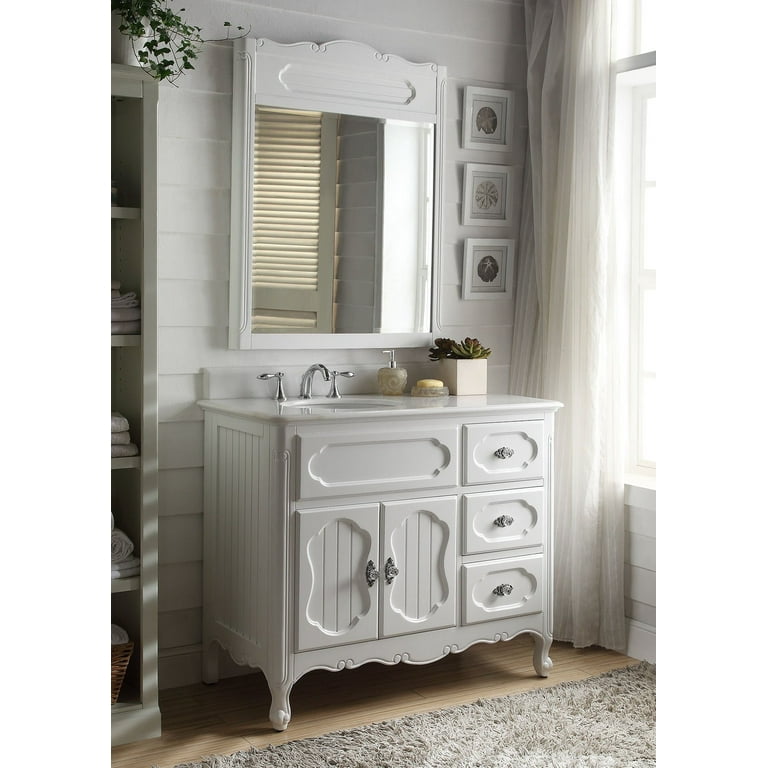The photograph depicts a bright, white bathroom featuring a central vanity. The vanity is adorned with crystal knobs on two doors and three accompanying drawers, all beneath a sleek white sink with a silver faucet and handles. Atop the vanity rests a silver soap dispenser, a dish with a bar of soap, and a small succulent. Above the vanity, a white-framed mirror is affixed against a backdrop of white wooden panels. To the right of the mirror are three small square pictures showcasing different seashells. Adjacent to this, a window with pulled-back, gauzy white curtains allows sunlight to flood the space. On the left side of the image, part of a shelf laden with neatly stacked towels is visible, capped with a plant in the top corner. Warm wooden floorboards and a beige rug complete the inviting scene.